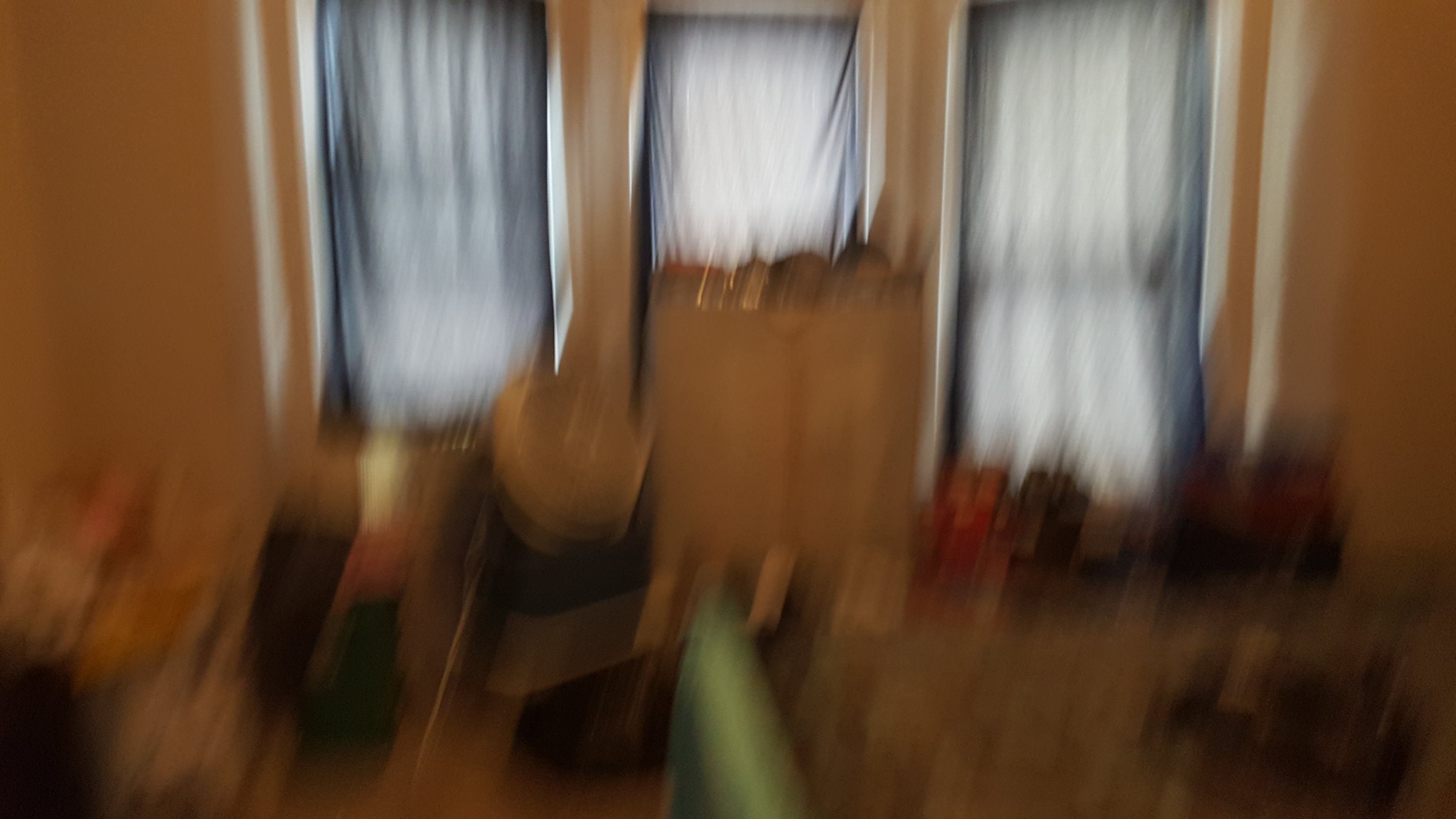A very blurry and underexposed image showcases an interior scene dominated by a medium brown tone. Three windows, partially obscured by drapes that appear to be white, though possibly gray due to poor lighting, are central to the composition. One window is partly uncovered, allowing white light to bleed through its edges. The foreground is jumbled and dark, with a blurry green object extending from the center of the bottom edge to about one-third of the image's height. The lower-left corner features an indistinct pile of items that vaguely resemble a table and chairs, though their details are lost in the blur and darkness. The overall lack of clarity suggests the photo was taken with a camera that moved during a long exposure in low-light conditions.